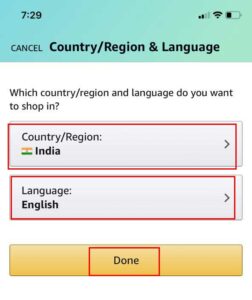In this screenshot, we observe a user interface screen with a prominent green gradient header displaying the number "729" in bold black letters. Directly below, there is text reading "Cancel, country/region, and language," also in black bold lettering. The top of the screen shows Wi-Fi signal bars and a nearly empty battery icon. 

The main section features a white background with bold black text asking, "Which country/region and language do you want to shop in?" Directly below are selections for "Country: India" with the corresponding Indian flag, and "Language: English." Each selection box has a noticeable red outline, indicating interactivity. To the right of these boxes, there is an arrow icon suggesting the ability to make a selection, followed by a yellow button at the very end of the interface, likely for confirmation or continuation of the process.